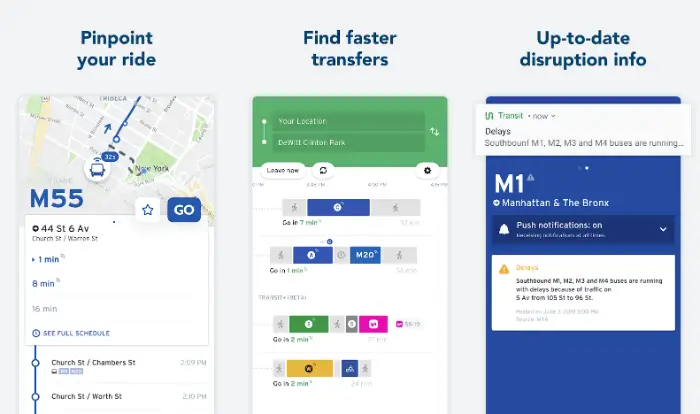Here's a detailed and cleaned-up caption for the described image:

---

This image showcases a mock-up of a mobile application, typical of those found on platforms like the Google Play Store or Apple App Store, designed to help potential users understand its interface and functionality. The mock-up is set against a light gray background and contains three distinctive rectangles, each representing how the app's screens might look on a smartphone.

At the top, there is a dark blue header with the text "Pinpoint Your Ride." Below this, Google Maps is displayed with a bus icon topped by a Wi-Fi symbol, indicating real-time tracking. The route is marked in dark blue, with "32S" for seconds. To the left, the route is labeled "M55". 

The first rectangle below the header is largely white. At the top right, a white square with a blue star sits beside a dark blue square featuring the word "Go" in white text. Beneath this, the address "44ST6AV" is written in black, with "Church Street CHURCHST / unreadable street name" in gray below it. It shows transit times: "1 minute" in blue with an arrow, followed by "8 minutes" and "16 minutes" in gray. An icon resembling a clock directs users to "See Full Schedule," indicating more detailed timing information. Specific scheduling information follows: "Church Street CHAMBERST" at 2:09 PM in gray, and "Church Street WORST STREET" at 2:10 PM.

A secondary section, topped with blue text saying "Find Faster Transfers," contains a green rectangle with a vertical white line flanked by two dots on the left and up-and-down arrows on the right. This section includes "YORK LOCATION," "DEWILLCLINTON PARK," and an interactive "Leave Now" button featuring a refresh symbol within a white circle. To the right, a gear icon appears for settings.

The third rectangle shows a gray horizontal layout: the left side displays a silhouette of a walking person, and the far right mirrors this with similar imagery. Centralized text reads "Go in 7 minutes," where "Go In" is black and "7 minutes" is green. Further details show varied icons and silhouettes: a white circle with a blue 'C', dark gray and mid-gray backgrounds with walking person icons, and wayfinding suggestions like "M20" bus stop identifiers in dark blue text. Additional time-related instructions ("Go in 1 minute," "Go in 2 minutes," etc.) are displayed in various colors (green, violet pink, orange), each accompanied by different icons.

This comprehensive mock-up gives users a clear idea of how they will navigate the app, track transit times and routes, find faster options, and access more detailed scheduling information.

---

This description covers the entire visual and functional aspects of the mock-up, clarifying the layout, color scheme, icons, and text to give a thorough and precise understanding.